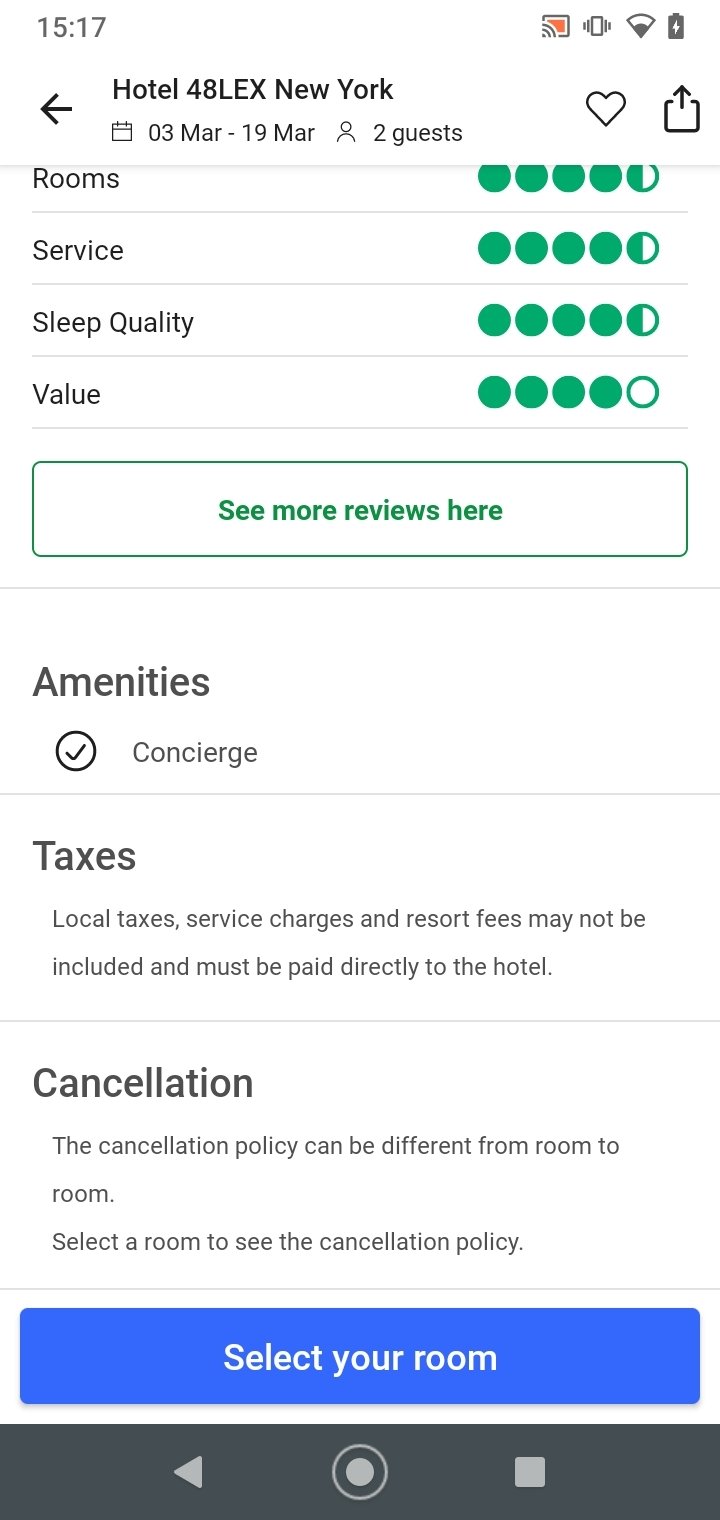This is a detailed screenshot of a cell phone screen. At the top left corner, the current time is displayed. On the right-hand side, various cell phone icons, such as signal strength, battery level, and notifications, are visible. Just a little below, the title of the page reads "Hotel 48 L.A.X. New York". Accompanying the title on the same bar, it indicates the dates "March 3rd to March 19th" and mentions that the reservation is for two guests.

Directly beneath the title bar, there are four distinct rows. Each row represents a different aspect of the hotel stay and includes a five-circle rating system colored in green:
- The first row is labeled "Rooms"
- The second row is "Service"
- The third one states "Sleep Quality"
- The fourth is marked "Value"

Each row’s rating is fully filled in, reflecting top ratings for all categories. 

Following these rows, there is a prominently displayed button stretching from left to right. The button has a green border with a white center, and the text "See More Reviews Here" is printed in green.

Below this button, there is a section dedicated to amenities, starting with "Concierge". The next section covers transportation options, titled "Taxi". Lastly, there is a "Cancellation" section down below that.